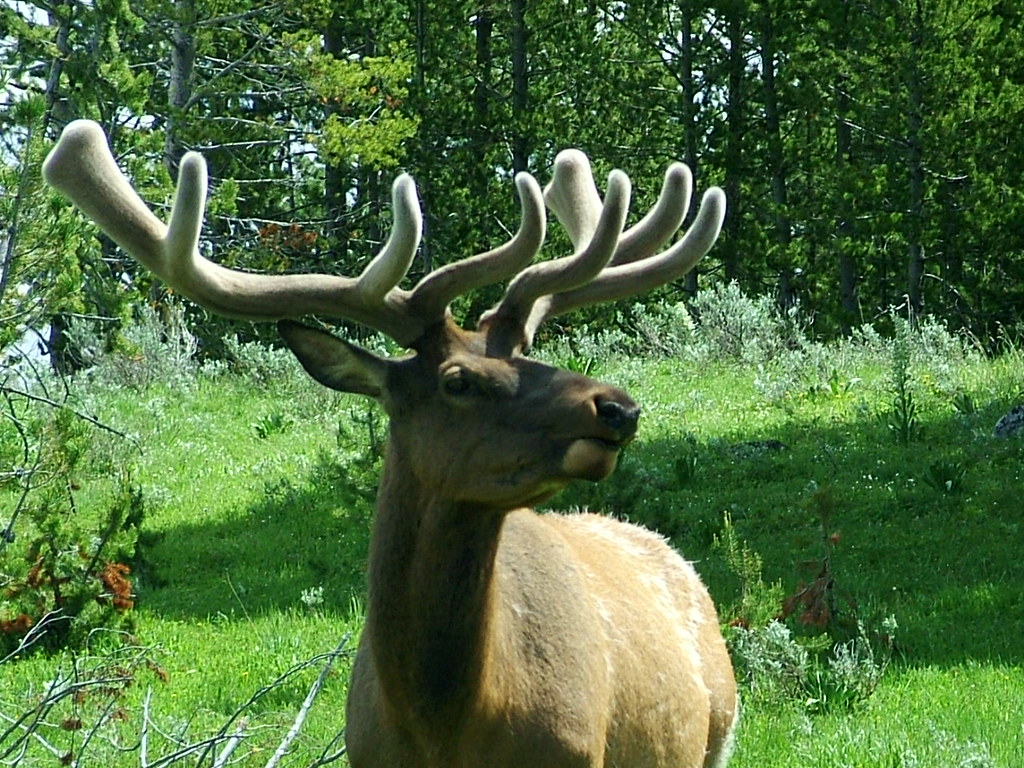The image captures a detailed and lifelike scene of a deer in what appears to be a digitally rendered forest. The background showcases tall, thin tree trunks with lush green leaves and patches of blue sky visible through the branches. In the middle and bottom sections of the image, a mix of short and tall grasses in varying shades of green, some with hints of white, covers the forest floor.

Dominating the foreground is a majestic brown deer, situated at the center of the frame. It is a close-up view, showing the deer from the neck and body upwards, with no legs visible. The deer sports large, fuzzy antlers, still wrapped in the mossy felt characteristic of spring. Each antler has four points. The deer's body faces the camera, while its head is turned to the right, revealing its right eye, black nose, and right ear.

Although the scene appears incredibly realistic, there is an almost mystical quality to the deer, suggesting it might have been digitally rendered and seamlessly integrated into the natural setting. Shadows cast to the left of the deer hint at a light source coming from the right side of the image. The palette of the photograph features predominantly green foliage, light brown hues from the deer, and subtle glimpses of blue sky, contributing to the serene woodland atmosphere.